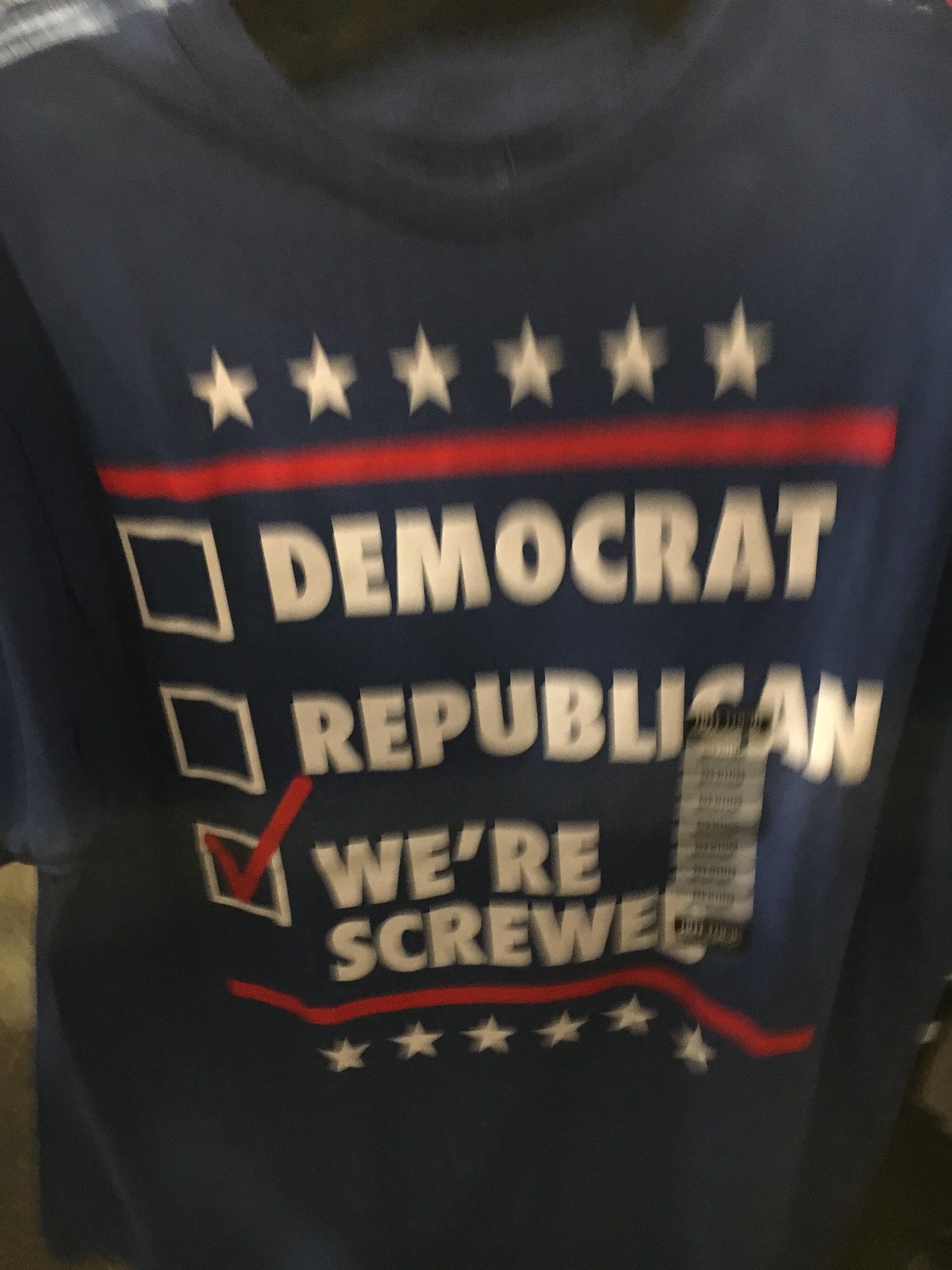In the image, we see a blue t-shirt hanging, presumably for sale. The design on the shirt features a series of six stars aligned across the top, followed by another set of six stars at the bottom. Between these sets of stars, there are three checkboxes. The top checkbox has the word "Democrat" written in large white letters next to it, while the middle checkbox has "Republican" similarly labeled. The bottom checkbox contains a red checkmark and is captioned with the phrase "We're Screwed" in large white letters. Additionally, there is a visible barcode present on the shirt.